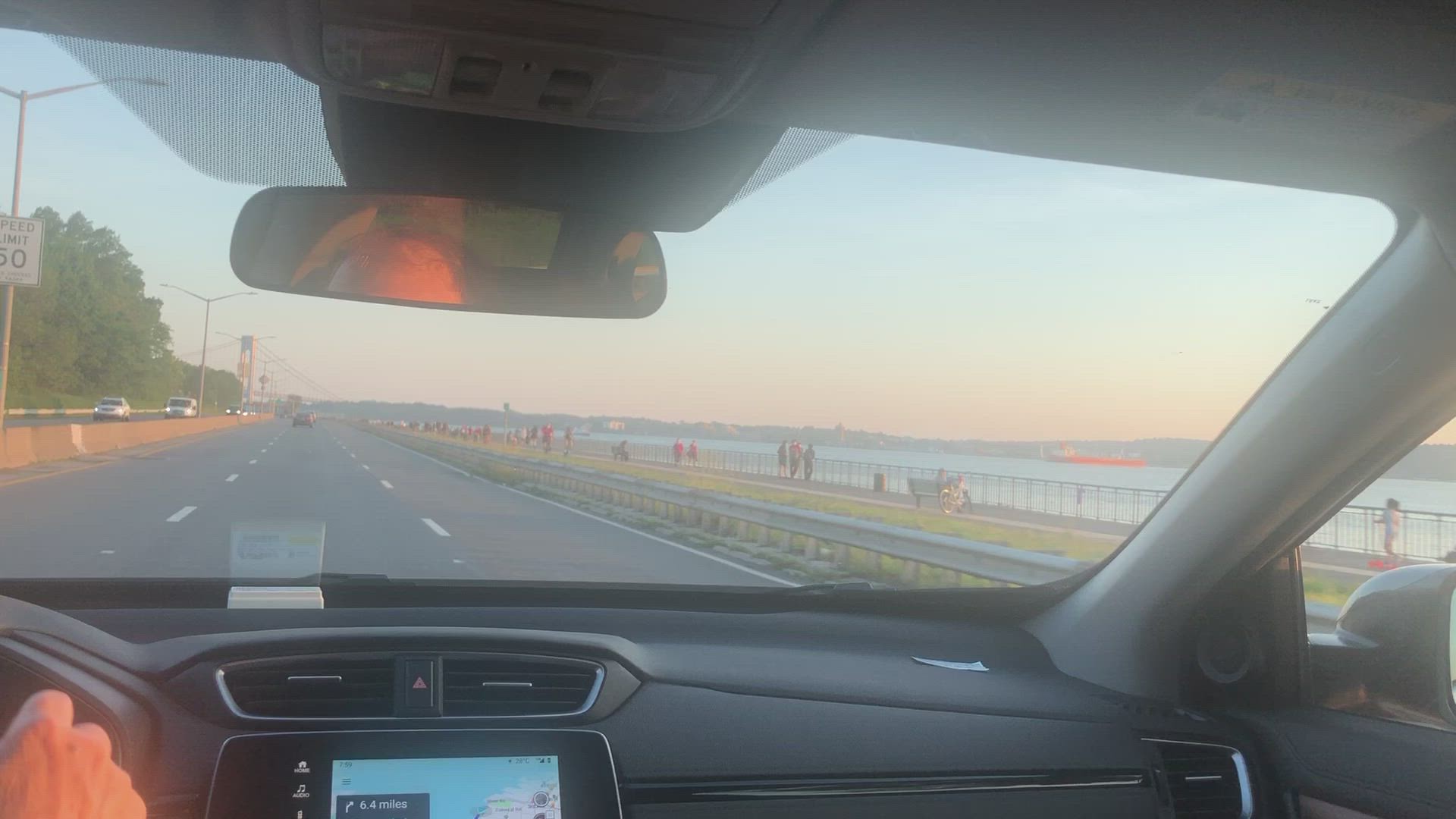This photograph captures an interior view from the backseat of a car driving down a three-lane highway at dusk. The foreground features a black dashboard with a navigation screen showing an upcoming turn in 6.4 miles, alongside the driver’s right hand gripping the steering wheel and the top of his bald head visible in the rear-view mirror. The asphalt road, distinctly marked with white lines, lies ahead. A concrete divider separates the oncoming traffic on the left, illuminated with headlights. Along the right, a gray guardrail leads to a wide expanse of green grass, followed by a cement walkway where various people are walking and sitting on benches, enjoying the waterside. The walkway is lined by a large fence for security. Beyond this, the scene opens up to a vast blue waterway, where a large red cargo ship can be seen in the distance. The far background reveals a range of low hills stretching across the horizon, and in the extreme distance, one section of the iconic Golden Gate Bridge is visible, adding a final touch of locale to this detailed scene.